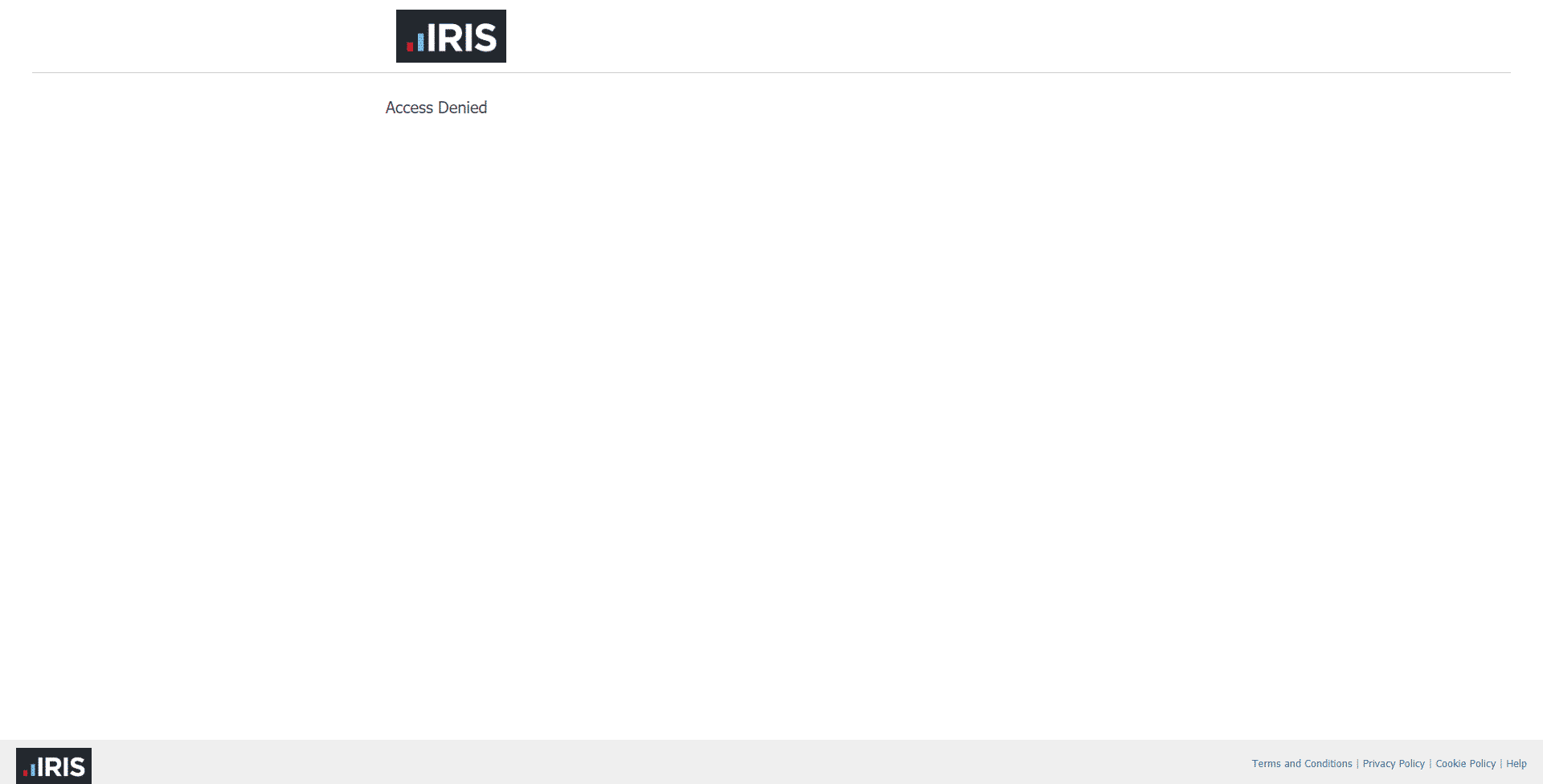This image depicts a clean, minimalist design with a predominantly white background. At the top, a thin, light gray horizontal line extends from left to right. Just right of the line's starting point is a distinctive black rectangular block. Inside this block, the word "IRIS" is boldly displayed in white, uppercase letters. To the left of the word "IRIS," there are two shorter vertical lines: the leftmost line is red and the line next to it is a bluish hue, neither extending as high as the word "IRIS". Directly below the black block containing "IRIS," in delicate gray font, the phrase "Access Denied" is printed, adding a sense of restriction or limitation. A similar black block featuring the word "IRIS" in white uppercase is also found at the bottom left of the image, embedded within a slim gray footer that runs horizontally across the bottom of the screenshot. The overall design is simple yet purposeful, using minimalistic elements to convey its message.